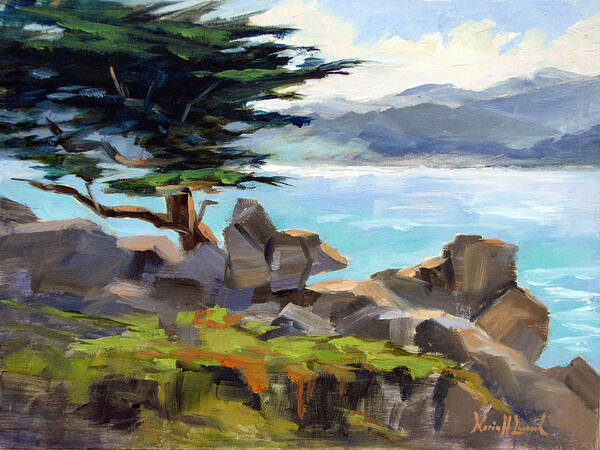In this evocative landscape painting, an idyllic scene unfolds with a single tree, akin to a bonsai, growing robustly on the edge of a rocky cliff. The cliff, composed of large, square boulders, boasts patches of green moss interspersed with orange growth, lending a vibrant touch. The foreground prominently features these rocks, some with dark brown trunks possibly holding the tree firm. Beneath the cliff, a serene body of green-hued water stretches out, perhaps suggesting a tropical lake. The water’s vibrant colors serve as a striking contrast to the grayish, rocky mountains in the background, which add a sense of depth and grandeur. Above, the sky is adorned with puffy white clouds against a light blue backdrop, enhancing the scene’s calm and tranquil atmosphere. At the bottom right corner, the artist's name is signed, appearing in orange, although partly indecipherable.